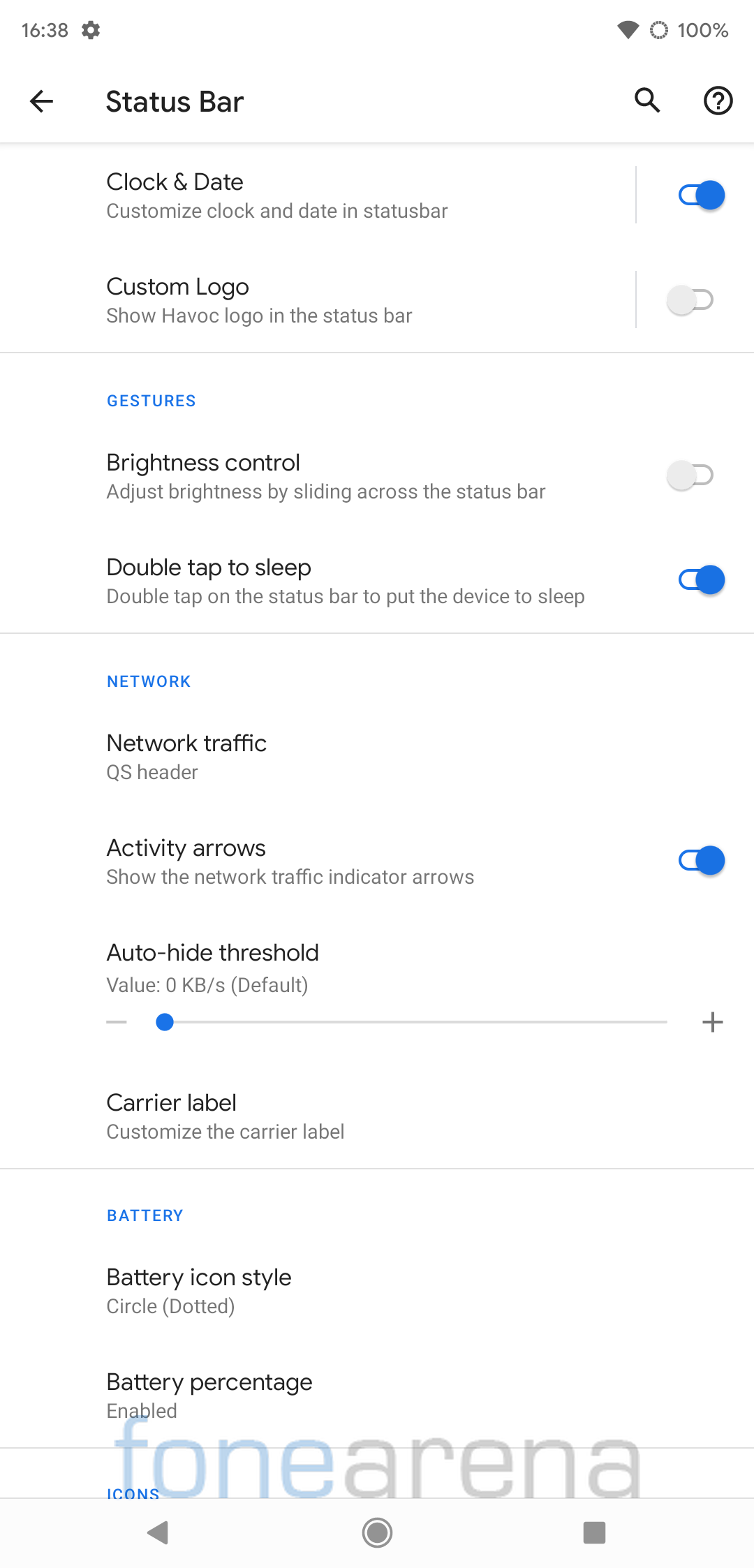The image is a screenshot taken from a cell phone, displaying a settings menu. At the top, the background is white, and it shows the time as "16:38" followed by a gear icon. To the right, there is a Wi-Fi symbol, and next to it, a circular icon resembling a donut with a dot in the center, indicating a full battery with "100%" written below it.

In the left section beneath the top area, there's a rightward-pointing arrow labeled "Status bar" in black text. Moving further right, there is a magnifying glass icon and a question mark enclosed in a circle.

Below this, a settings option reads "Clock and Date," with a subheading "Customize clock and date in status bar." This setting has been activated, as indicated by a blue slider button. When the slider is toggled off, a white dot appears on the left, but in this case, the slider is blue and positioned to the right. 

Another setting for a "Custom logo" is turned off. Further down, options for "Gestures" are listed, where the "Brightness control" is disabled, the "Double tap to sleep" feature is enabled, and the "Activity arrows" setting is also enabled. The page contains various other settings as well.